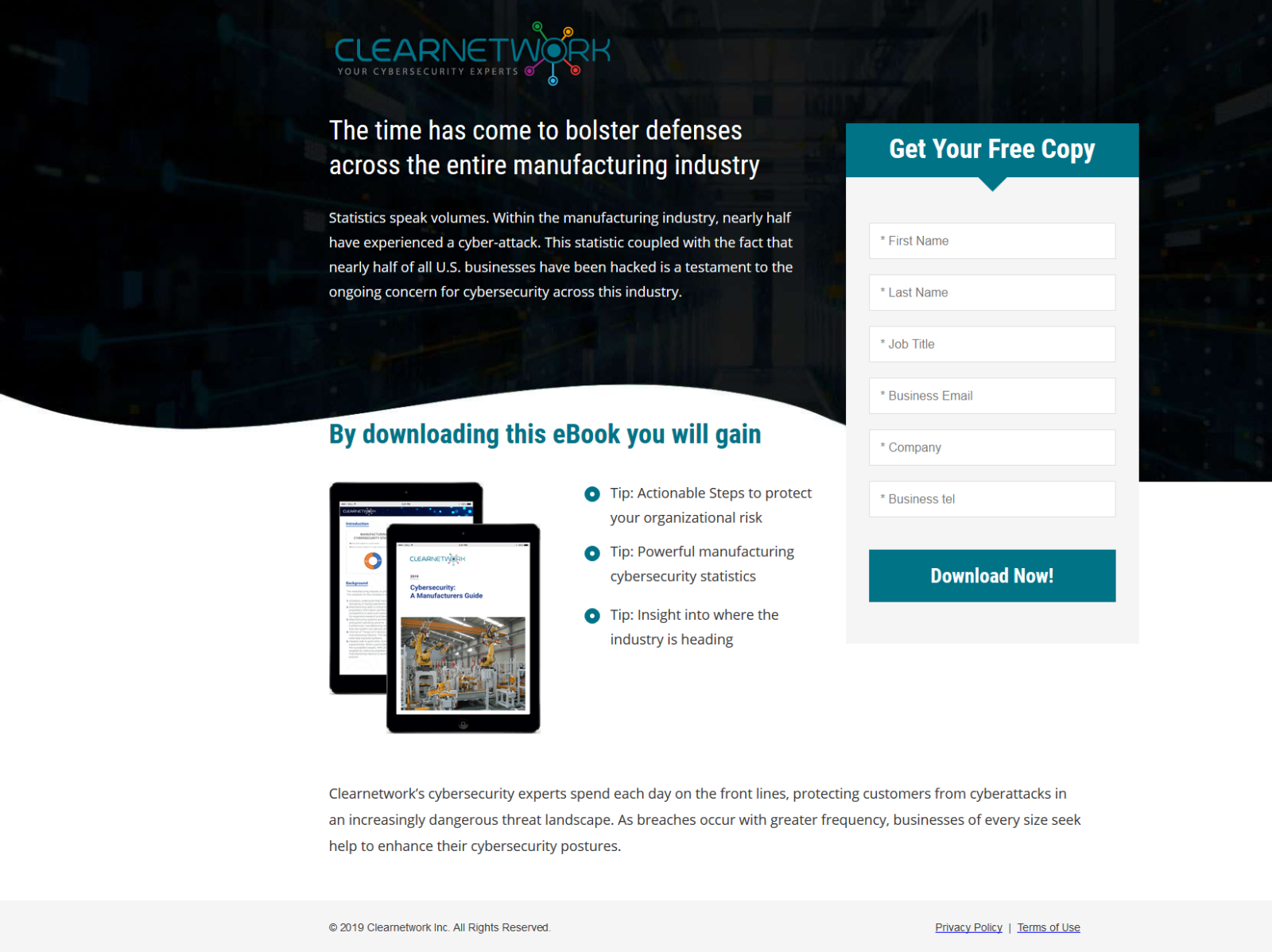The webpage from Clear Network emphasizes the critical importance of bolstering cybersecurity across the manufacturing industry. Highlighting the urgency, it underscores that nearly half of the industry has experienced cyber-attacks, reflecting a similar trend in businesses across the United States. This statistic underscores the persistent and growing concern regarding cybersecurity in the manufacturing sector.

The site prominently features a call-to-action with a "Get Your Free Copy" dialog box on the right side. This box, outlined in blue with a white background, includes fields for entering personal and professional information such as First Name, Last Name, Job Title, Business Email, Company, and Business Telephone. A "Download Now" button below these fields invites users to access a free eBook.

The eBook promises to provide valuable insights through bullet points, including tips and actionable steps to protect organizations, powerful manufacturing cyber statistics, and an overview of where the industry is heading. The page features two images of an iPad, one showing the cover titled "Cyber Security Manufacturer's Guide" and the other displaying a pie chart, illustrating detailed cybersecurity data.

Underneath, the text highlights Clear Network's expertise, mentioning that their cybersecurity experts work daily on the front lines to protect customers from increasingly frequent and dangerous cyber threats. The page also notes that breaches are becoming more frequent, pushing organizations of all sizes to seek enhanced cybersecurity measures.

The bottom-right corner of the page contains links to the Privacy Policy and Terms of Use, noting that the content is © 2019 Clear Network, Incorporated, all rights reserved.